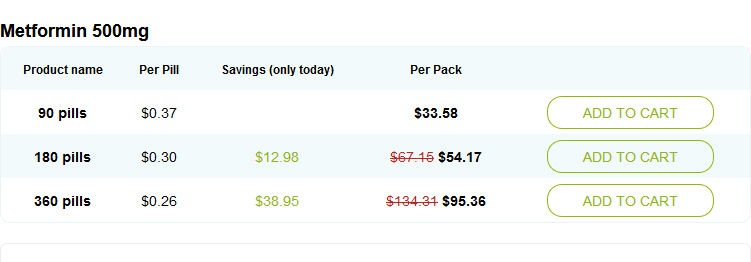In this color, landscape-format screenshot, a person browses online for purchasing Metformin 500 mg. The image reveals three distinct product options available for the consumer. The choices include packs of 90, 180, and 360 pills. The 90-pill pack is priced at $33.58, the 180-pill pack offers a better rate at $54.17, and the 360-pill pack provides the best value at $95.36. A breakdown of the cost per pill reveals that buying in larger quantities decreases the price per pill: $0.37 for the 90-pill pack, $0.30 for the 180-pill pack, and $0.26 for the 360-pill pack. This detailed pricing information aids the viewer in determining the most cost-effective option for purchasing Metformin 500 mg online.